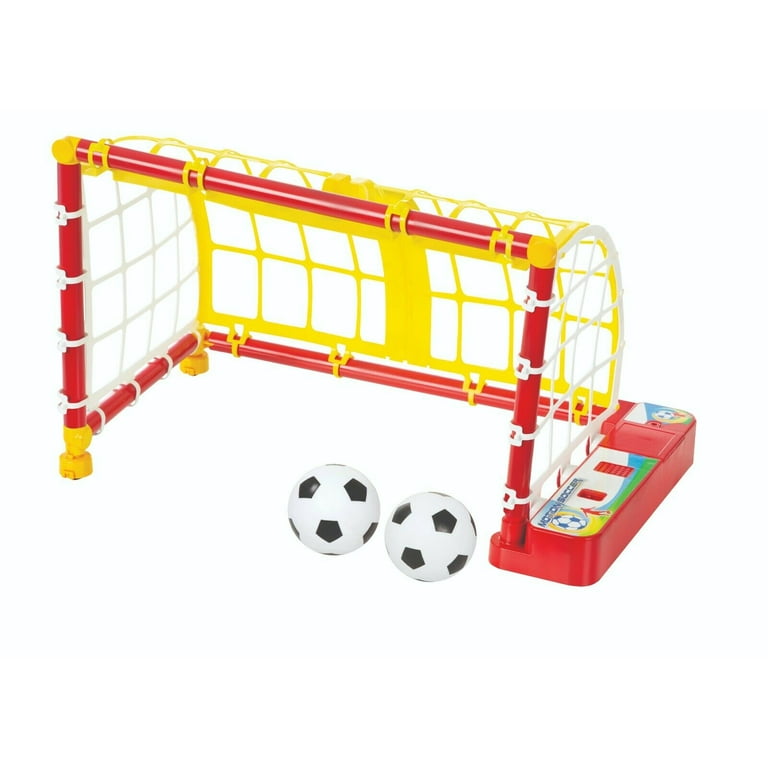This image is of a toy soccer playset designed for young children, likely around five to six years old. The playset is showcased on a solid white background in a marketing-style photograph. It features a colorful soccer goal net with a red frame that forms a horizontal rectangle. The net itself is bright yellow, with white netting on the sides. On the right side of the frame, there is a red plastic rectangular area with graphics and logos, including the words "Motion Soccer." This section also includes a red switch and a depiction of a small red-outlined soccer player on a green field, indicating some interactive element and a possible battery compartment.

In front of the net, there are two small toy soccer balls, both white with classic black pentagon markings, characteristic of traditional soccer balls. The overall aesthetic of the set, with its vibrant colors and plastic construction, suggests it is a fun and engaging toy for children, resembling something from Fisher-Price.